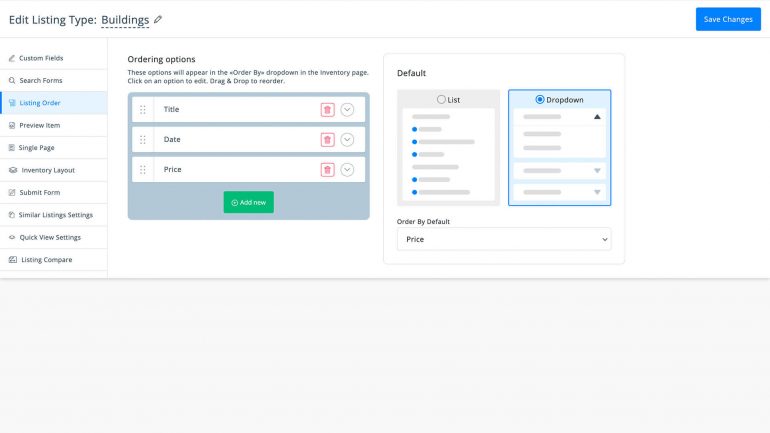The image displays a computer screen with an interface for editing building listings. The title "Edit Building Listings" is prominently written in black text, with the word "Buildings" being underlined and in a very dark blue ink. Next to the word "Buildings" is a small pencil icon, suggesting an edit function.

On the left side of the screen is a vertical column of selectable options. The options are listed in the following order: Custom Fields, Search Forms, Listing Order, Preview Item, Single Page Inventory Layout, Submit Form, Similar Listing Settings, Quick View Settings, and Listing Compare. Each option is accompanied by a small icon that visually represents its function, such as a magnifying glass next to "Search Forms". The third option, "Listing Order," is highlighted in blue with a light blue background, while the other options remain in black text on a white background.

The right side of the interface is divided into two sections. The first section, "Ordering Options," provides a description and includes categories for Title, Date, and Price, along with a green "Add New" button. The second section, labeled "Default," contains two selectable options: "List" and "Dropdown," with "Dropdown" currently highlighted in light blue. Below these sections, the space is populated by gray lines and a few triangle icons, indicating placeholder information yet to be filled in.